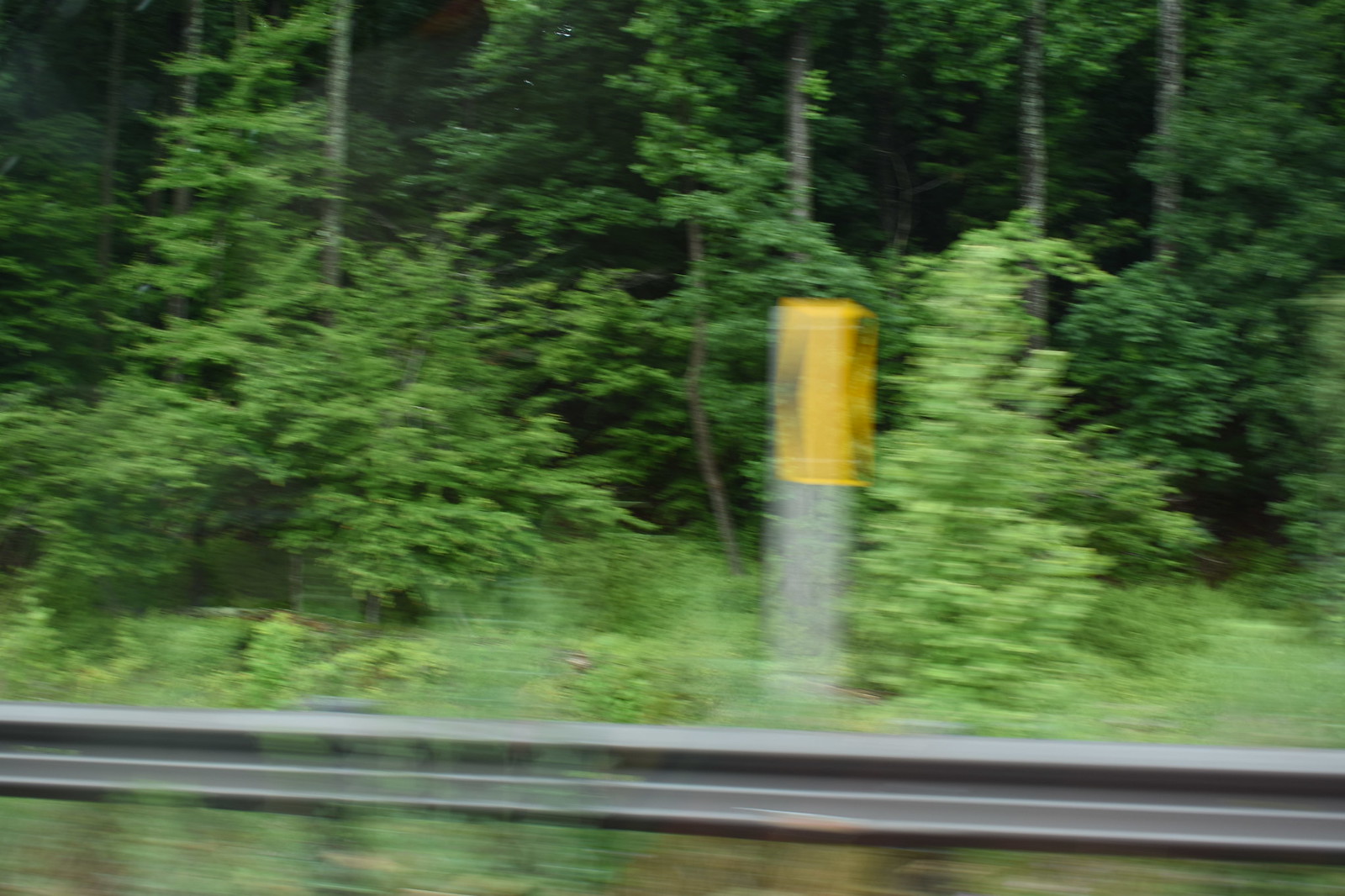The photograph, taken from inside a moving car, is slightly blurry, suggesting a high speed. In the foreground, there's a metal guardrail running parallel to the road. Just beyond the guardrail, a road sign stands out; it has a yellow top segment featuring black arrows pointing to the left. The scene is lush with greenery, marked by dense vegetation and vibrant grass. A mix of shorter and very tall, full trees extends into the distance, forming a thick, shaded forest that recedes into the background. The overall composition gives an impression of driving quickly through a verdant, forested landscape.